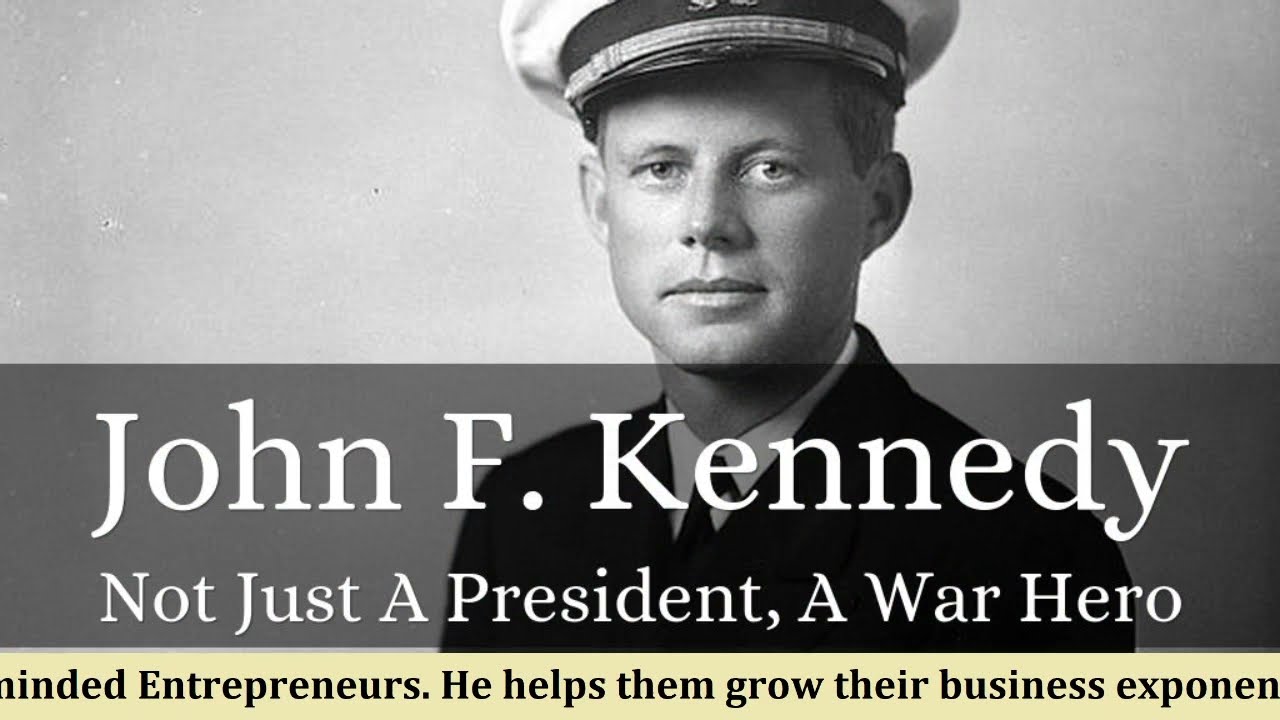This black and white banner features a photograph of a young John F. Kennedy, dressed in a military suit and wearing a white captain's hat with a black bill, likely from his time in the Navy. The image bears the bold white text "John F. Kennedy" at the top, followed by the tagline "Not just a president, a war hero" in smaller, yet still prominent, white font. Below, a partially obscured yellow and white banner begins with "minded entrepreneurs," continuing with, "he helps them grow their business exponentially." The background of the text area is a muted gray, bringing focus to the image of Kennedy, evoking his legacy as both a revered leader and a distinguished war hero.